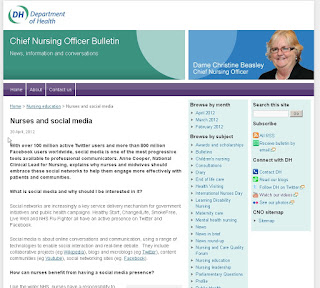This image depicts the Department of Health's Chief Nursing Officer Bulletin, which serves as a platform for news, information, and discussions pertinent to the nursing profession. The focal point of the image is Dame Christine Beasley, the Chief Nursing Officer, who is featured prominently with her short blonde hair and glasses against a plain blue background, likely added via a green screen technique.

The bulletin includes an article titled "Nurses in Social Media," presumably authored by Dame Christine Beasley, though the text remains largely unreadable due to the blurriness of the image. The bulletin allows users to navigate articles by their posting dates, arranged by months such as April, March, and February. There are multiple hyperlinks embedded within the bulletin, directing to various external websites, as well as essential sections like Home, About, and Contact Us. However, the overall blurriness and small size of the image obscure additional details.